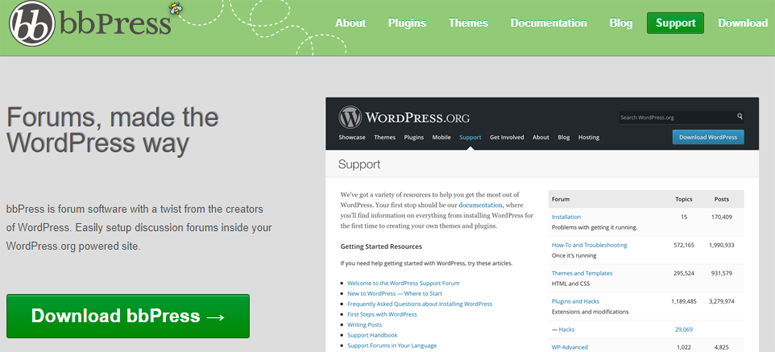Here is a cleaned-up and detailed caption of the described image:

---

This image depicts a website interface with a structured layout. In the upper left corner, there is a circular logo featuring a white border and a black interior with the white letters "BB" inscribed. Adjacent to the logo, the text "BB Press" appears in black lettering, accompanied by a small cartoon image of a bee fluttering on a green background.

Below this header, there are several navigation options including "About," "Plugins," "Themes," "Documentation," "Blog," "Support," and "Download." The "Support" option stands out as a green button with white text, whereas the other options are presented in white text on a green background.

In a gray-shaded section of the page, the phrase "Forums made the WordPress way" is prominently displayed. This is followed by a brief description stating, "BB Press is forum software with a twist from the creators of WordPress. Easily set up discussion forums inside your WordPress.org powered site." Positioned below this description is a green button labeled "Download BB Press."

On the right side of the image, there is a portion showcasing the WordPress.org site with options such as "Showcase," "Themes," "Plugins," "Mobile," "Support," "Get Involved," "About," "Blog," and "Hosting." Additionally, a message indicates the availability of various resources aimed at aiding WordPress users. It advises that "Your first step should be our documentation," which provides information on everything from the initial installation of WordPress to the creation of custom themes and plugins. Below this, there are links to "getting started resources."